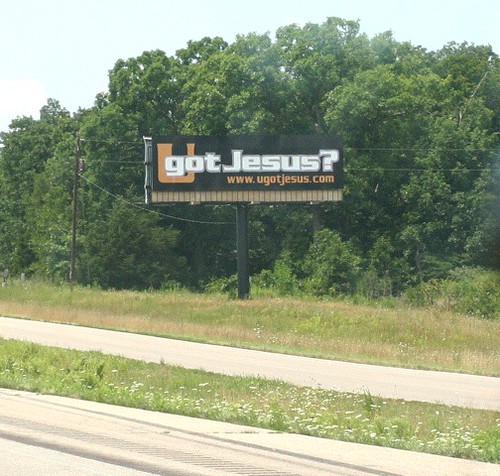This photograph captures a moment on the side of a highway, likely shot from a passenger seat facing slightly forward. A feeder road is visible at an angle in the background. The scene is dominated by a large roadside sign mounted on a thick, black, round pole. The sign prominently displays a message in two parts: the letter "U" in tan against a black backdrop, followed by "Got Jesus?" in bold white text. Beneath this, a website URL, www.yougotjesus.com, is clearly legible. Surrounding the sign are numerous trees and telephone or electrical lines, all set against a clear, sunny summer day's sky.